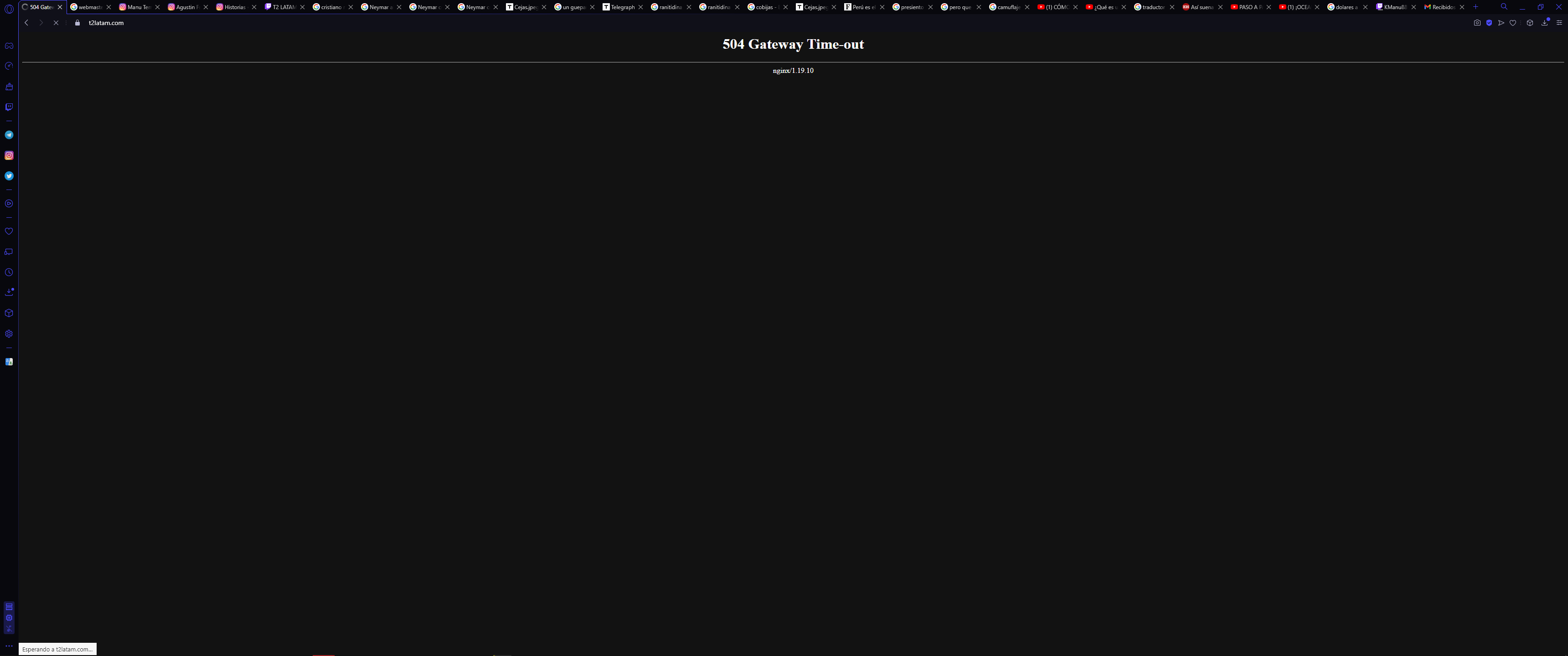The image shows a desktop screenshot of a website attempting to be accessed through what appears to be the Chrome web browser. However, the browser interface is unusual, featuring a strange vertical menu bar or settings that are unclear. The user is trying to load "T2LATAM.com" but receives a "504 Gateway Timeout NGINX/1.19.10" error message. At the bottom of the browser, there is a Spanish phrase "Esperando," indicating an attempt to load the site unsuccessfully.

The horizontal bar at the top displays various icons for platforms such as Twitch, Instagram, Twitter, LinkedIn, YouTube, and Reddit, alongside other icons like a heart, a monitor, a time download (with a notification indicator), a box, a hyphen, and one resembling an old Apple Finder menu.

There are numerous open tabs across the top—more than 13 different Google searches, three Instagram tabs, one Twitch tab, several indistinguishable tabs with a 'T' favicon, and around four YouTube video tabs. Overall, the browser has an excessive number of open tabs, likely over 20, contributing to the cluttered appearance and possibly the website loading issues.